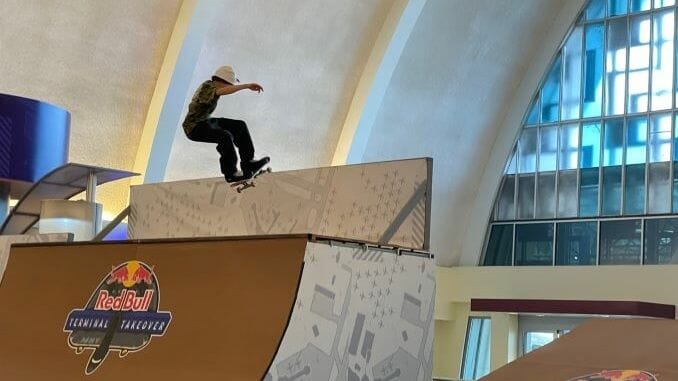This detailed color photograph captures an indoor skate park housed within an expansive building resembling a Quonset hut, characterized by its semi-circular, perfectly rounded roof and white curved walls. Featuring prominently in the image is a skateboarder in mid-air, showcasing his skills on a light brown half pipe. The skateboarder, dressed in long pants, a dark short-sleeve shirt, and a white helmet that possibly has a camera mounted on it, is captured in action, making it impossible to see the floor. In the background, a large stained glass window allows natural light to filter into the space, complementing the overall luminous environment. The facility is clearly sponsored by Red Bull, as indicated by the visible Red Bull logo on the half pipe, alongside the text "Terminal Takeover." The descriptive scene illustrates both the architectural uniqueness of the skate park and the dynamic energy of the skateboarding activity within it.